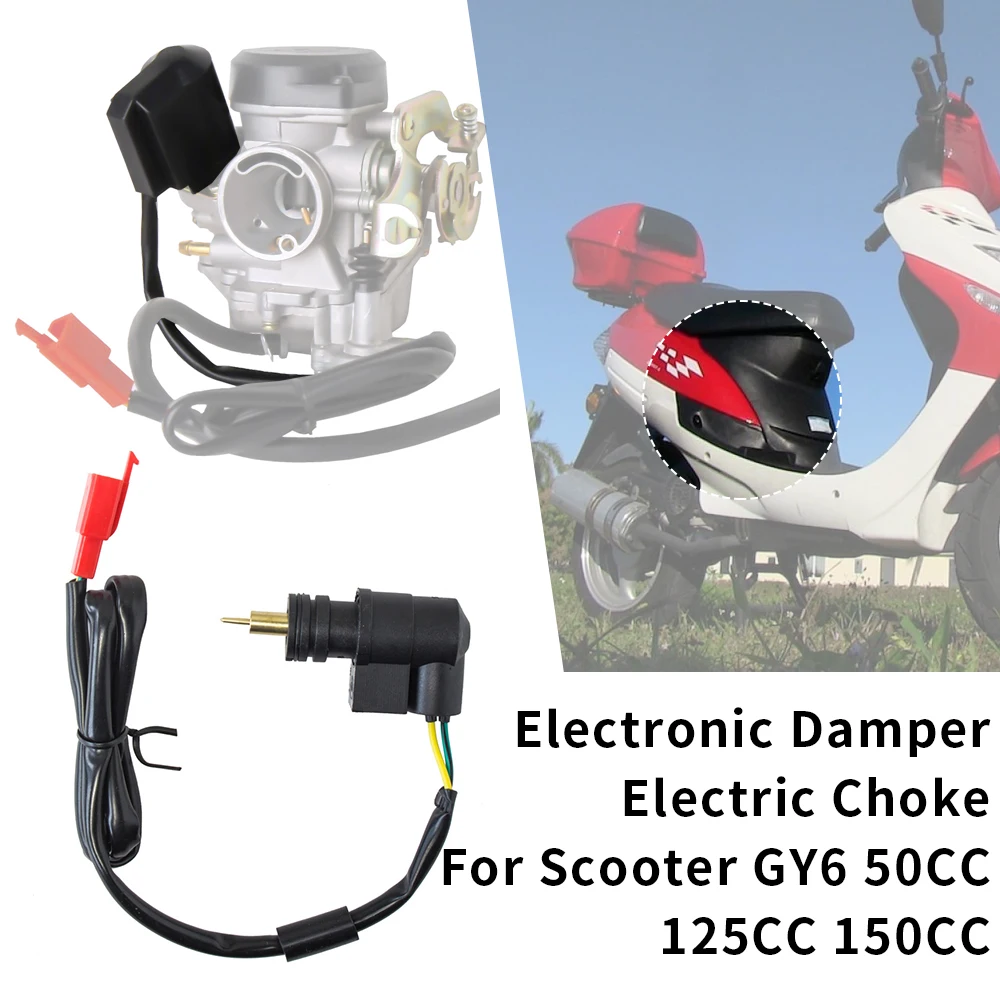This image prominently features a red, white, and black gas-powered adult scooter. The main focus is emphasized by a highlighted circle that draws attention to a specific mechanical component on the scooter. This featured component, located on the left side of the image, is a gray and silver electronic damper or electric choke with black cords and a distinct red plug. One of the cords extends to a black plug with a gold connector. The background of the image has a white overlay, and additional text on the bottom right corner clarifies the part as an "electronic damper, electric choke for scooter GY6, 50cc, 125cc, 150cc." The image is designed to illustrate the exact location and detail of the part in relation to the scooter.